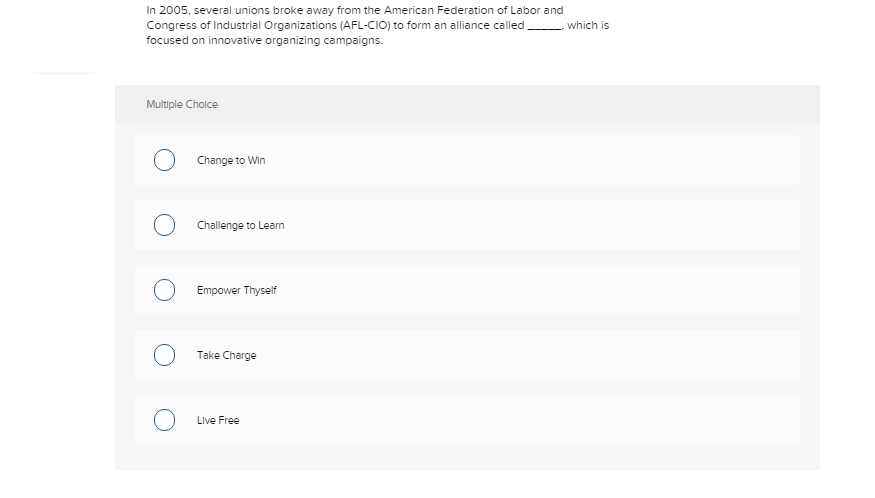The image features a minimalist design with a white background and centered text. At the top, it reads: "In 2005, several unions broke away from the American Federation of Labor and Congress of Industrial Organizations (AFL-CIO) to form an alliance called Blank, which is focused on innovative organizing campaigns." Below this is a gray box labeled "Multiple Choice." Within this box are five white, unchecked boxes arranged in a vertical column, each accompanied by a different option. The options are: "Change to Win," "Challenge to Learn," "Empower Thyself," "Take Charge," and "Live Free." The image is simple and direct, focusing on the multiple-choice format with the intent of selecting the correct answer.